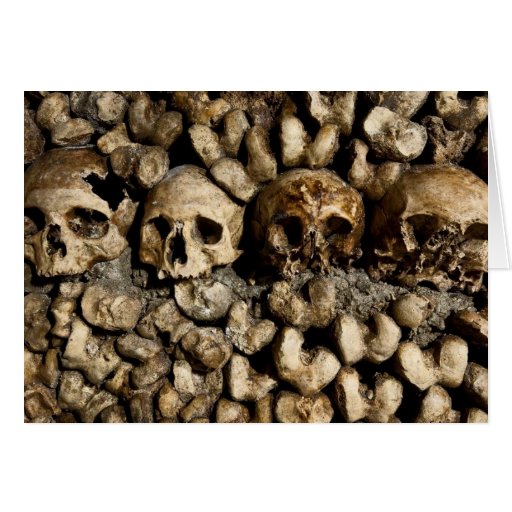The image shows a tightly focused view of a wall made of bones, with four human skulls prominently positioned in a row near the center. Surrounding these skulls are numerous leg and arm bones, likely femurs, that form the top and bottom sections of the wall. The scene is set against a background of dirt and mud, giving it an ancient and eerie appearance. The skulls themselves display varying degrees of damage and discoloration; the two on the left are lighter in color, while those on the right are darker and dirtier, possibly suggesting a layer of dark brown dirt or mud smudging them. The skull on the far left has a large hole, and the one on the far right has significant damage to the lower facial region. The image evokes a sense of being in a catacomb, such as the Paris Catacombs, where human remains are meticulously arranged, evoking a somber and historic atmosphere. The color palette is dominated by shades of white, off-white, brown, black, and gray, enhancing the gritty and somber mood.